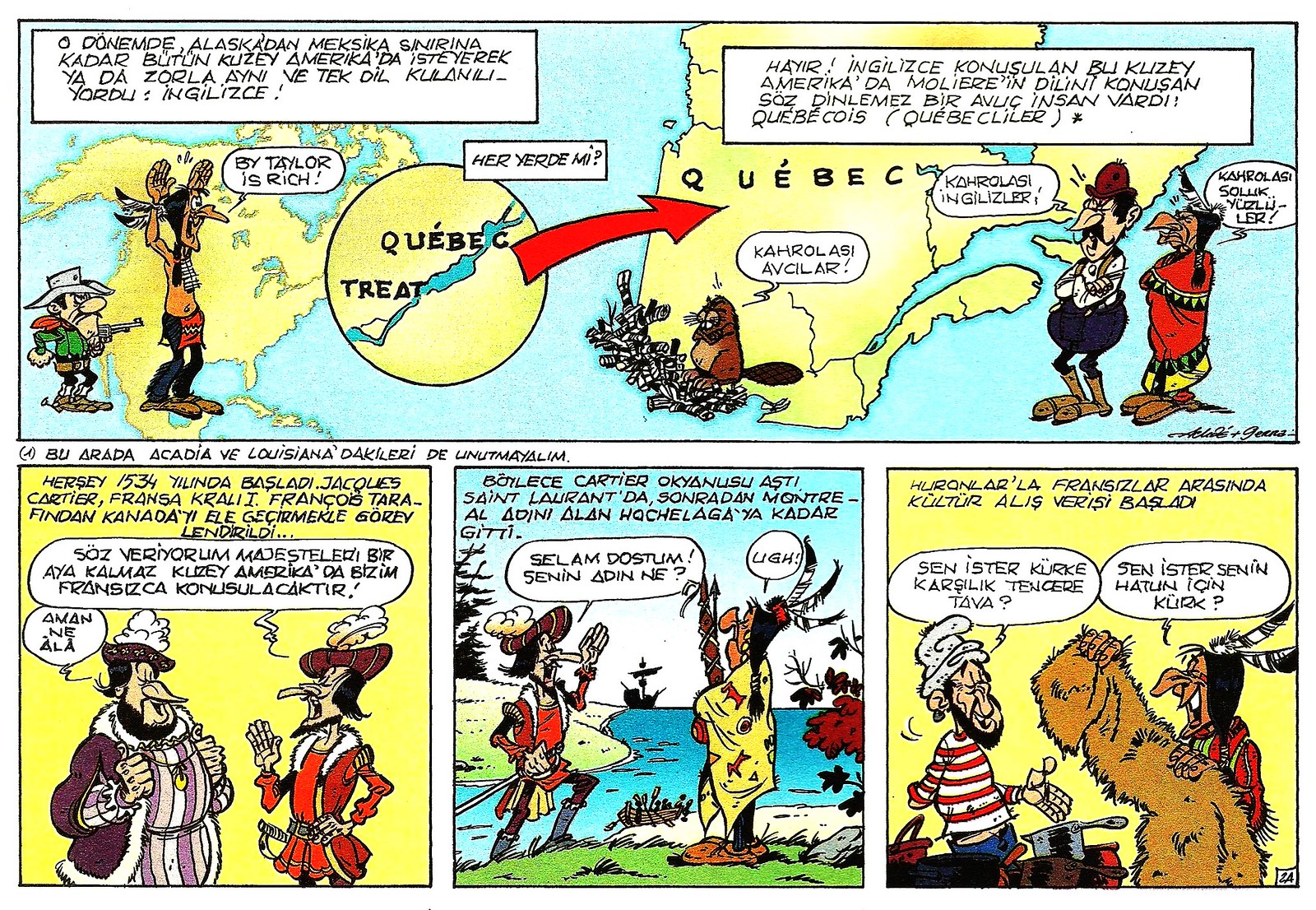This detailed comic strip, divided into four panels with a prominent long horizontal rectangle at the top, features a satirical depiction of historical events and diverse cultural interactions. The text within the comic appears to be in a foreign language, potentially French, making it challenging to decipher exact dialogue. Dominating the scene are playful caricatures of cowboys and Indigenous peoples, reflecting a blend of historical and cultural references.

In the first scene, a cowboy is holding a gun to the back of an Indigenous man, who has his arms raised in surrender, with the phrase "Quebec Treat" prominently displayed in a circle. A red arrow points toward the word "Quebec," suggesting a connection to the location. The Indigenous man is dressed in traditional attire with a red robe and a single feather.

The comic also includes a map of Quebec, surrounded by quotes and dialogue presumably expressing conflicts and negotiations about the land. Colorful art showcases settlers and Indigenous people in a dispute, with visual elements like a ship in the background symbolizing colonial arrivals. The hand-drawn cartoons emphasize the satirical nature of the piece, highlighting the tumultuous interactions and historical tensions over centuries.

Overall, this comic strip uses vivid visual storytelling to satirize and critique public events and cultural encounters, featuring figures that resemble Indigenous people, cowboys, and possibly early European settlers in Quebec.